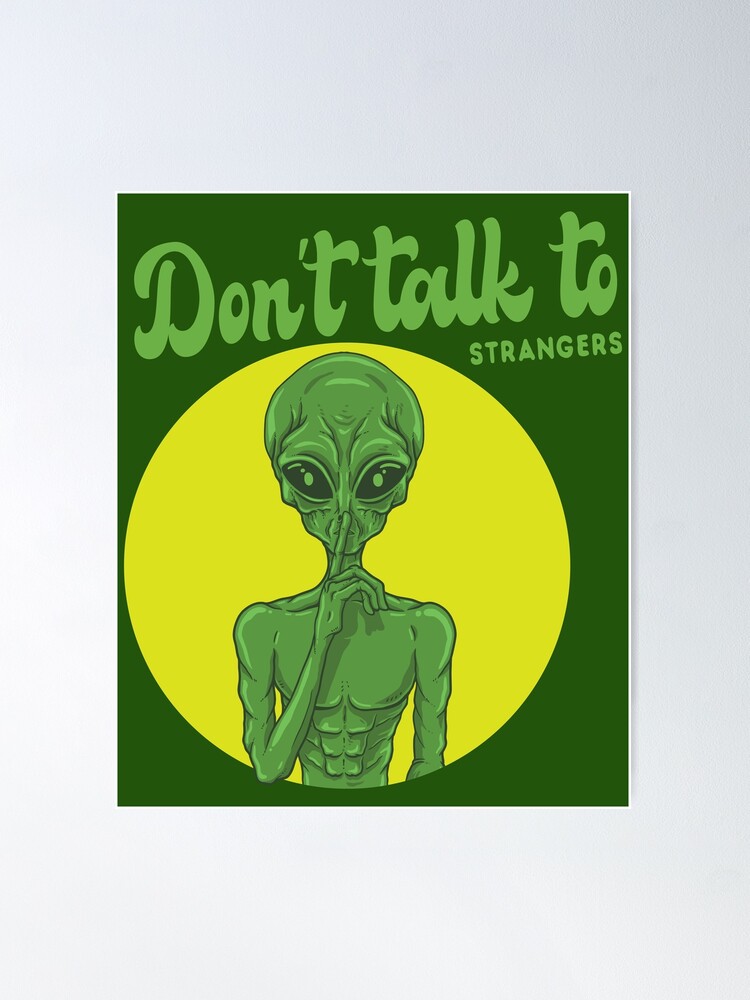This image is a cute and eye-catching public service announcement poster advising both kids and adults not to talk to strangers. Set against a white background, the central green poster features a whimsical cursive typography that reads "Don't talk to strangers," with "strangers" written in a smaller, non-cursive font. The green background is contrasted by a large yellow circle housing a peculiar, skeletal, and green alien figure. This alien, reminiscent of E.T. with its exaggeratedly large head and big black eyes, strikes a pose with one of its long, skinny fingers held up to its lips in a shushing gesture. Emphasizing the message, the alien's muscled, abs-clad torso is visible, though the rest of its body remains unseen. The playful yet cautionary tone and the vibrant color scheme make this poster a standout, effectively grabbing attention while conveying the important message to avoid talking to strangers.